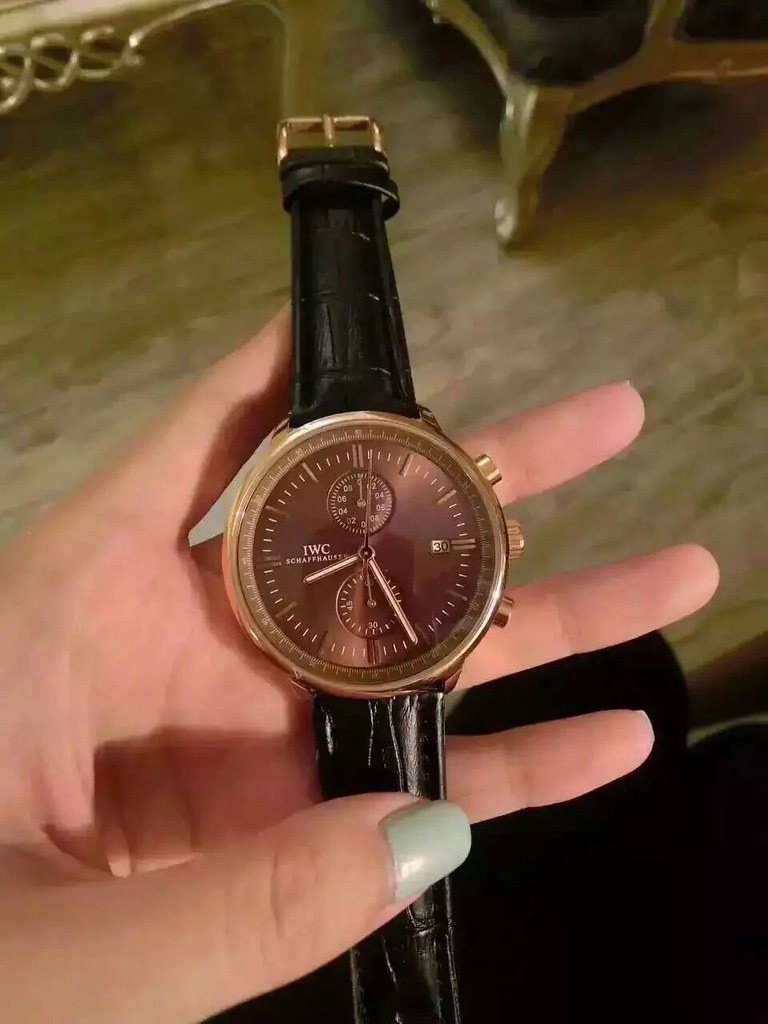A white woman is holding a stylish wristwatch in her hand. The watch features a black leather band and a round face with a glass cover, rimmed in gold. The face of the watch has a distinctive bronze, copper-like color, reminiscent of a new penny. Instead of traditional numbers, the watch has sleek lines marking the hours, minutes, and even seconds. The time displayed on the watch is 8:25. The woman's nails are painted a light blue, contrasting elegantly with the timepiece. The background of the image reveals a wooden floor, adding a touch of warmth to the scene.